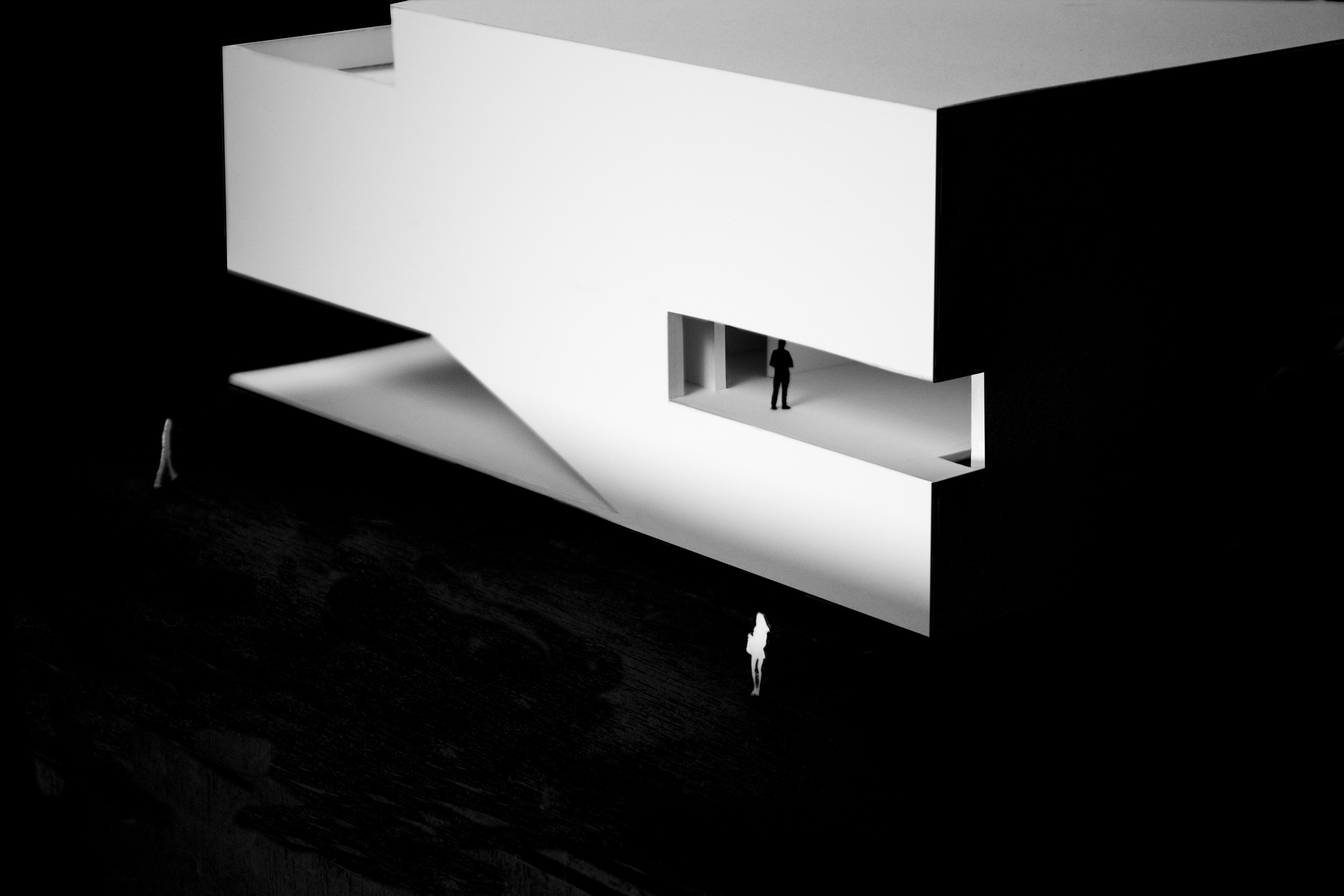The image is a striking 3D illustration or designed artwork showcasing a modern, white building prominently set against a completely dark background, creating a vivid contrast. The building includes a white roof and facade with some sides entirely black. A wing juts out at the second-floor level, forming a covered space, and features an open air hallway with open doors. Within this hallway, a black silhouette of a person can be seen. Below this, at ground level, there are two small white figures, likely a woman dressed in white and another indistinct figure, both appearing as if they are walking toward the building. The stark black-and-white contrast of the image, along with its precise architectural lines and the presence of the tiny figures, gives it the appearance of a photo negative or a detailed architectural replica.